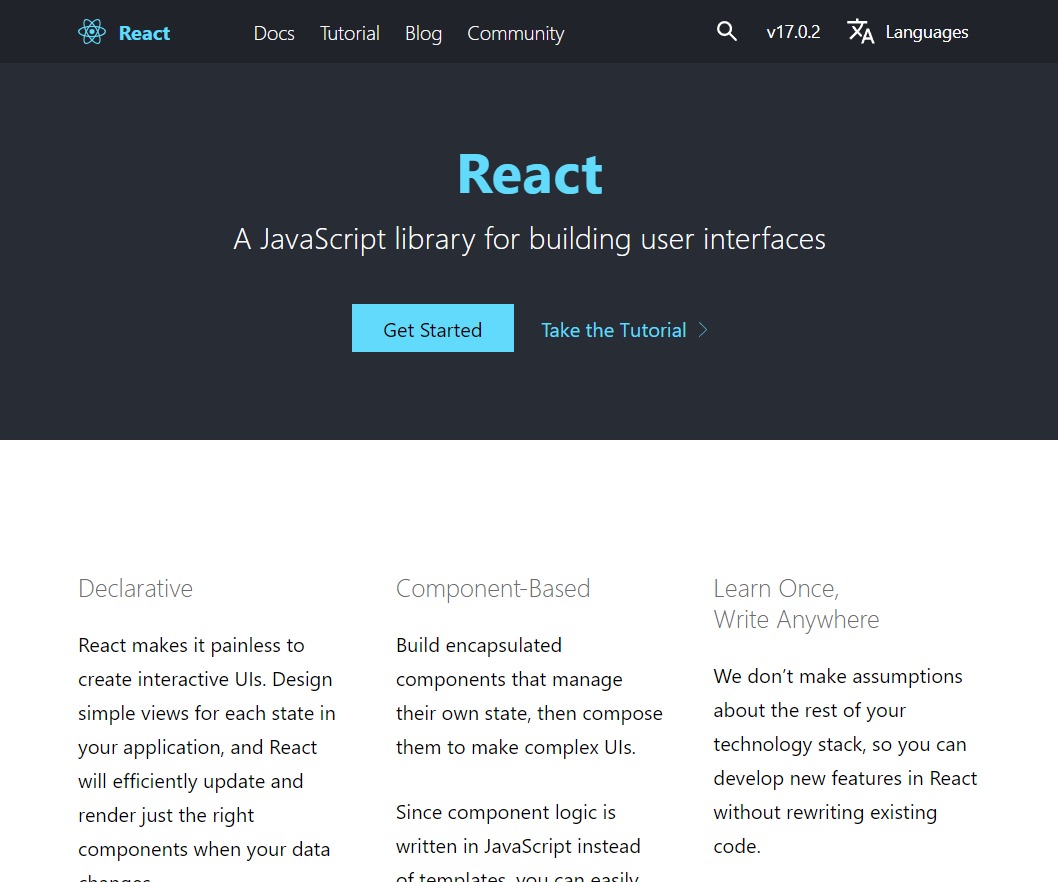The image is a screenshot of a web page with a dual-tone background. The bottom half features a white background, while the top half is a dark bluish-gray. The very top border is black. On the upper left corner, the word "React" is prominently displayed in a turquoise blue font, with a logo to its left resembling atomic orbits, indicative of atoms and electrons.

Spanning across the top in white font, items on the menu include "Docs," "Tutorial," "Blog," and "Community." Towards the right side, there's a search icon represented by a little circle with an extended line, and in the far right corner, the word "Languages" appears, suggesting the availability of multilingual options.

In the center of the dark bluish-gray background, the word "React" is again displayed in a vibrant turquoise blue, followed by the description "A JavaScript library for building user interfaces" in white font. Beneath this text, there's a prominent turquoise blue rectangular button labeled "Get Started" in dark blue font. Below this button, the phrase "Take the Tutorial" appears in blue font against the dark background.

The bottom half of the image, with the white background, is structured into three columns. Each column has a title and a brief description beneath it. The left column is titled "Declarative," the middle column is labeled "Component-Based," and the right one reads "Learn Once, Write Anywhere." Each section provides a succinct introduction to the features users can expect from React.